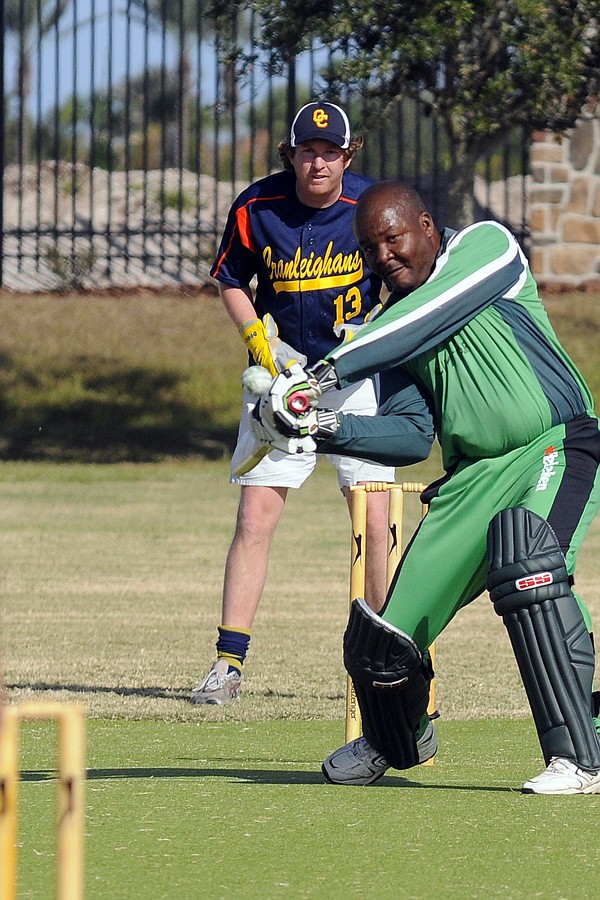In this vibrant color photograph, two men are engaged in a lively game of cricket on a sunny day, against the backdrop of a lush green grass field. The central figure is a bald, slightly chubby black man, around 35 to 40 years old, captured mid-swing with his cricket bat as the ball approaches. He is dressed in a distinctive green uniform with a teal-dark midnight green stripe on the pants, and padded gray shin guards extending over his knees. The uniform features a red star, suggesting sponsorship by Heineken. Behind him stands a Caucasian player from the opposing team, identified by the yellow number 13 on his dark blue jersey adorned with red lettering, which appears to read "Cran Lay-ins." This player also sports a blue and white hat emblazoned with "OC" or "QC." The scene is framed by a wrought iron fence and a stone pillar made of various stones cemented together, with a hint of blue sky and a tree in the background.